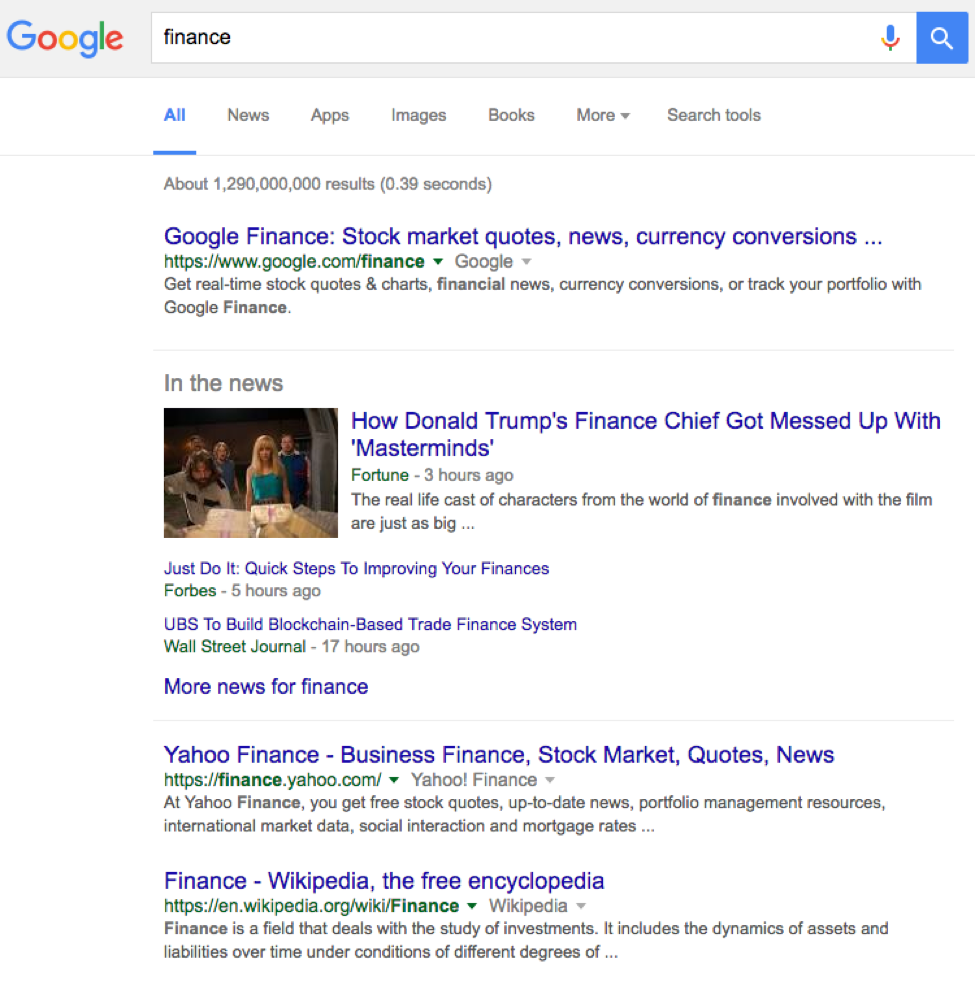The image depicts a Google search results page for "Google Finance." The search bar at the top features the Google logo, with "finance" typed into the search field. Adjacent to the search bar are icons for a microphone and a blue square containing a magnifying glass.

Below the search bar, there are navigation tabs labeled "All," "News," "Apps," "Images," "Books," "More," and "Search Tools." The "All" tab is highlighted in blue, indicating an active selection.

The results summary indicates approximately 1,290,000,000 results delivered in 0.39 seconds. The primary result is a link to Google Finance, described as offering real-time stock quotes and charts, financial news, currency conversions, and portfolio tracking.

Prominently featured in the news section is a headline about Donald Trump's fiancée's chief getting involved with "masterminds" from the world of finance, suggesting a connection with real-life characters from a film. Other highlighted articles include practical steps to improving personal finances, UBS's initiative to build a blockchain-based trade finance system, and additional finance news.

Moreover, the page includes a mention of Yahoo Finance as a source for business finance, stock market quotes, and news.